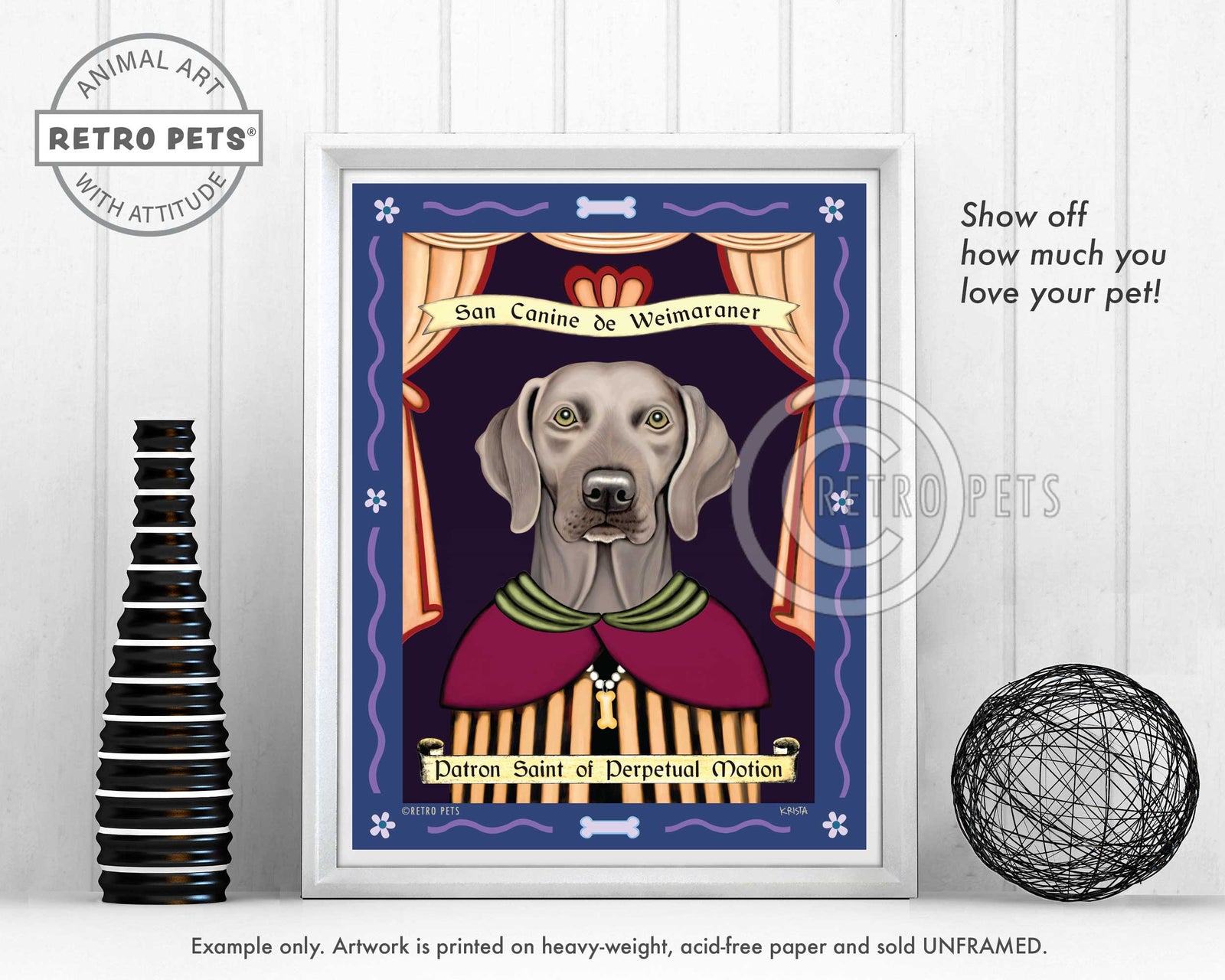The image is a detailed advertisement for animal-themed artwork under the brand "Retro Pets with Attitude." At the top center, a circular logo reads "Animal Art" and "With Attitude," encapsulating the creative and lively theme. The centerpiece of the image features a white wood-framed picture of a gray Weimaraner dog, dressed in a burgundy cape and a dog bone necklace, epitomizing playful nobility. Above the dog, a banner proclaims "San Canine de Weimaraner," while below, the text reads "Patron Saint of Perpetual Motion," adding a humorous saintly characterization. The background consists of white wooden slats, giving a rustic feel, and the image is adorned with a decorative blue border with a pet bone motif. To the left of the framed picture, there's a black vase with white lines and a textured design, complemented by a black, wic-like ball on the right. This composition not only showcases the artwork but also emphasizes how it can add a charming touch to pet lovers' décor.